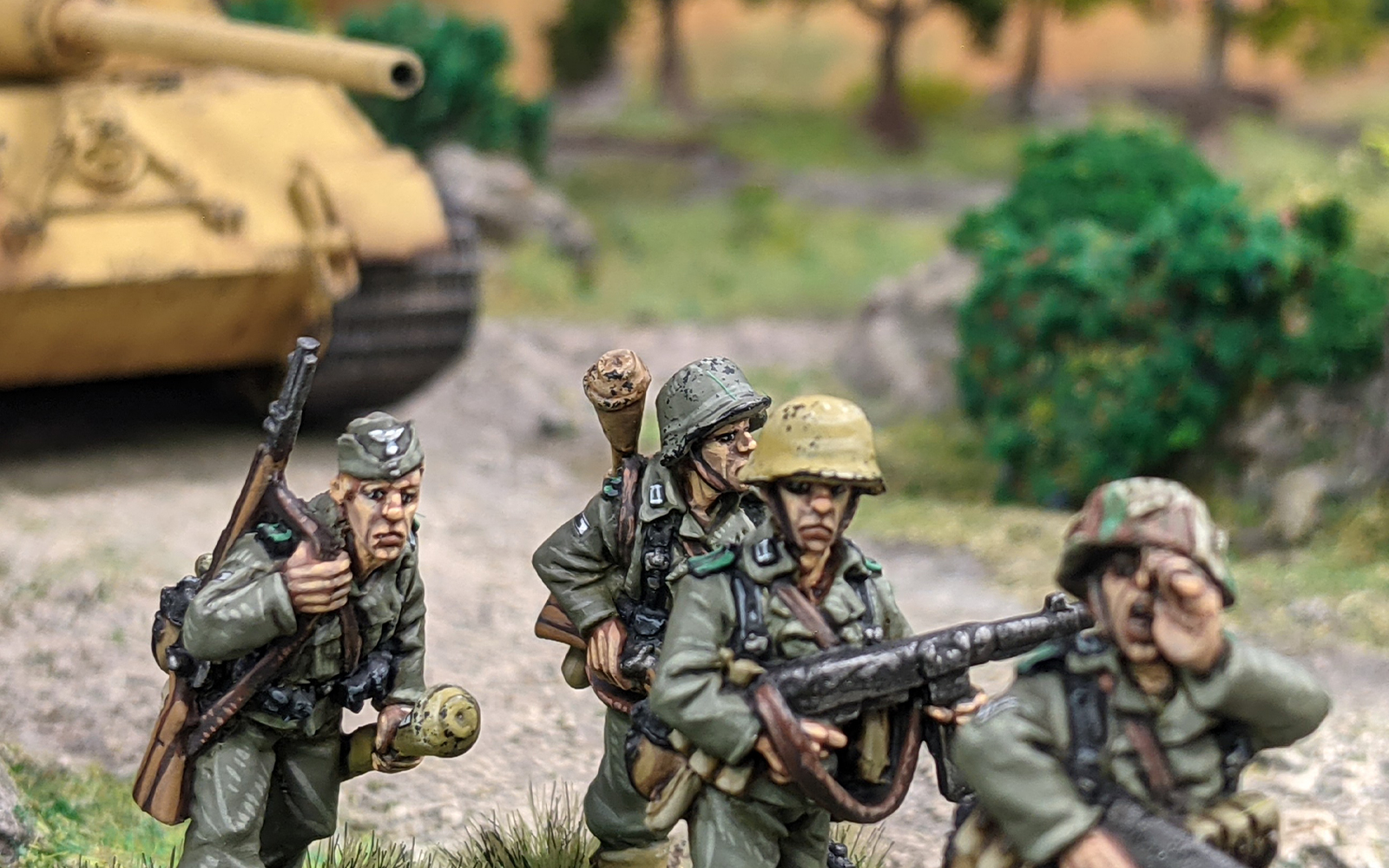The image displays four intricately crafted toy soldiers, seemingly made of clay or a similar material, positioned in front of a yellow toy tank. These soldiers are clad in traditional military gear, including plain green uniforms mixed with hints of browns and yellows, and are equipped with helmets.

From left to right:
1. The first soldier on the left is slightly apart from the group, carrying a rifle over his shoulder and holding something round in his hands. His face appears stern and focused.
2. The second soldier, positioned middle-left, is holding his rifle and appears to be closely observing his surroundings.
3. The third soldier, middle-right, is in front of the second soldier and is similarly engaged with his rifle, looking attentive and braced for action.
4. The soldier on the far right has his right arm supporting his rifle while his left hand is raised to his face, possibly signaling or shouting commands.

In the background, a yellow tank follows behind these soldiers, its long nozzle pointed ahead. The scene is set on a terrain adorned with grass, green bushes, and additional elements suggesting a diorama backdrop, complete with rocks and trees. The overall impression of the models gives a detailed and animated portrayal of a military unit progressing with purpose.